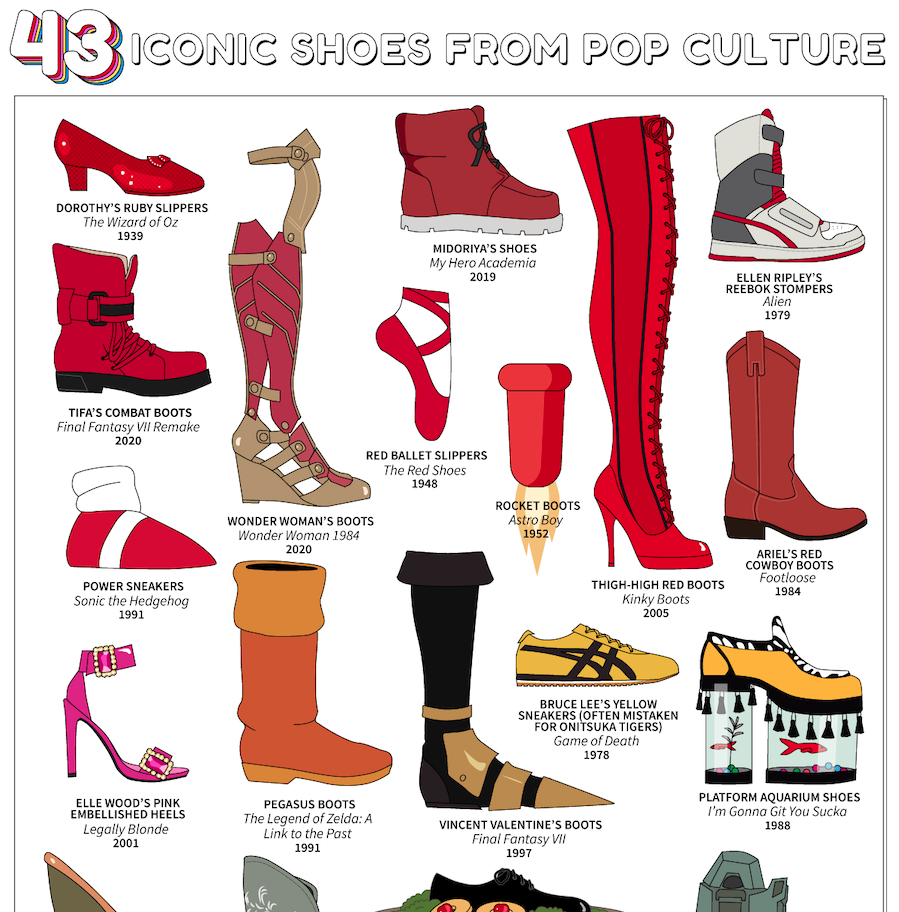A detailed poster featuring 43 iconic shoes from pop culture on a white backdrop, with illustrations of various famed footwear arranged in neat rows. At the top of the poster, the text reads "43 Iconic Shoes from Pop Culture". Each shoe is depicted facing right and vividly colored. The notable pairs include Dorothy’s Ruby Slippers from "The Wizard of Oz" (1939) in sparkling red, prominently positioned at the top left, while Ellen Ripley’s Reebok Stompers from "Alien" (1979), a two-tone gray high-top boot with red stripes, sits at the top right. Other memorable footwear includes Tifa’s Combat Boots from "Final Fantasy 7 Remake" (2020), featuring robust design elements; Wonder Woman’s Boots from "Wonder Woman 1984" (2020), characterized by their tall, strappy structure in red and tan; the whimsical Platform Aquarium Shoes from "I’m Gonna Get You Sucka" (1988), with clear glass fish tanks for soles; and the striking Thigh High Red Boots from "Kinky Boots" (2005). Each shoe entry is labeled with the character's name, the title, and the year of the movie or game, creating a comprehensive and nostalgic visual compilation of iconic footwear in pop culture history.